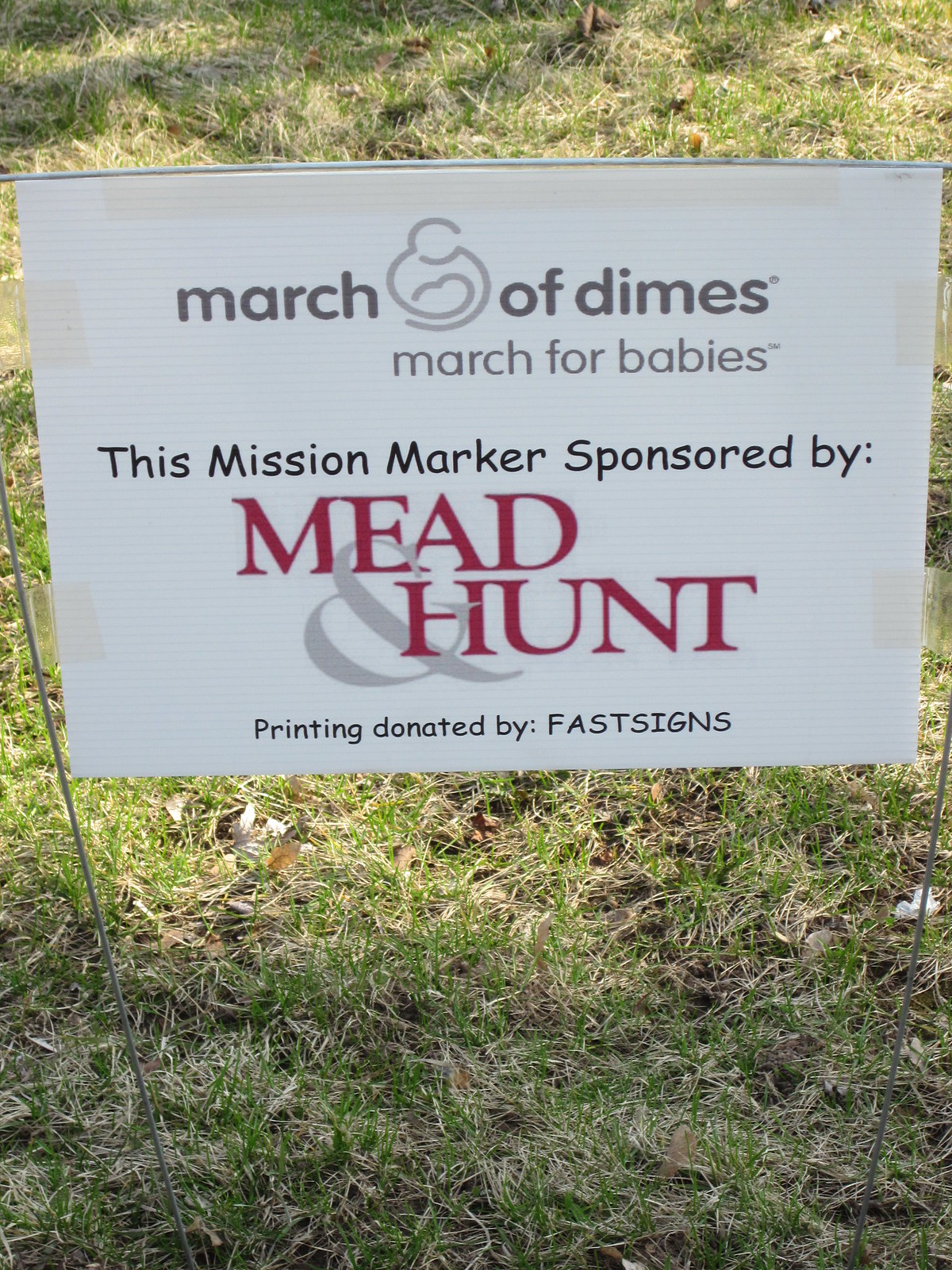The image captures a white sign staked into the grass using a thin metal wire. The sign contains multiple lines of text and a logo. In descending order, the text reads: "March of Dimes" on the first line, "March for Babies" on the second line. Between "March" and "of" there is a logo resembling a simplistic, stick-figure woman with a baby in her stomach, represented by two circles and a squiggly line outline. The third line states, "This Mission Marker Sponsored By," followed by "Mead & Hunt" in bold red font, with the ampersand symbol (&) in gray. Below, the final line says, "Printing Donated by Fast Signs" in capital letters. The grass where the sign is staked appears patchy and scattered with leaves, suggesting it is either late fall or mid-summer.